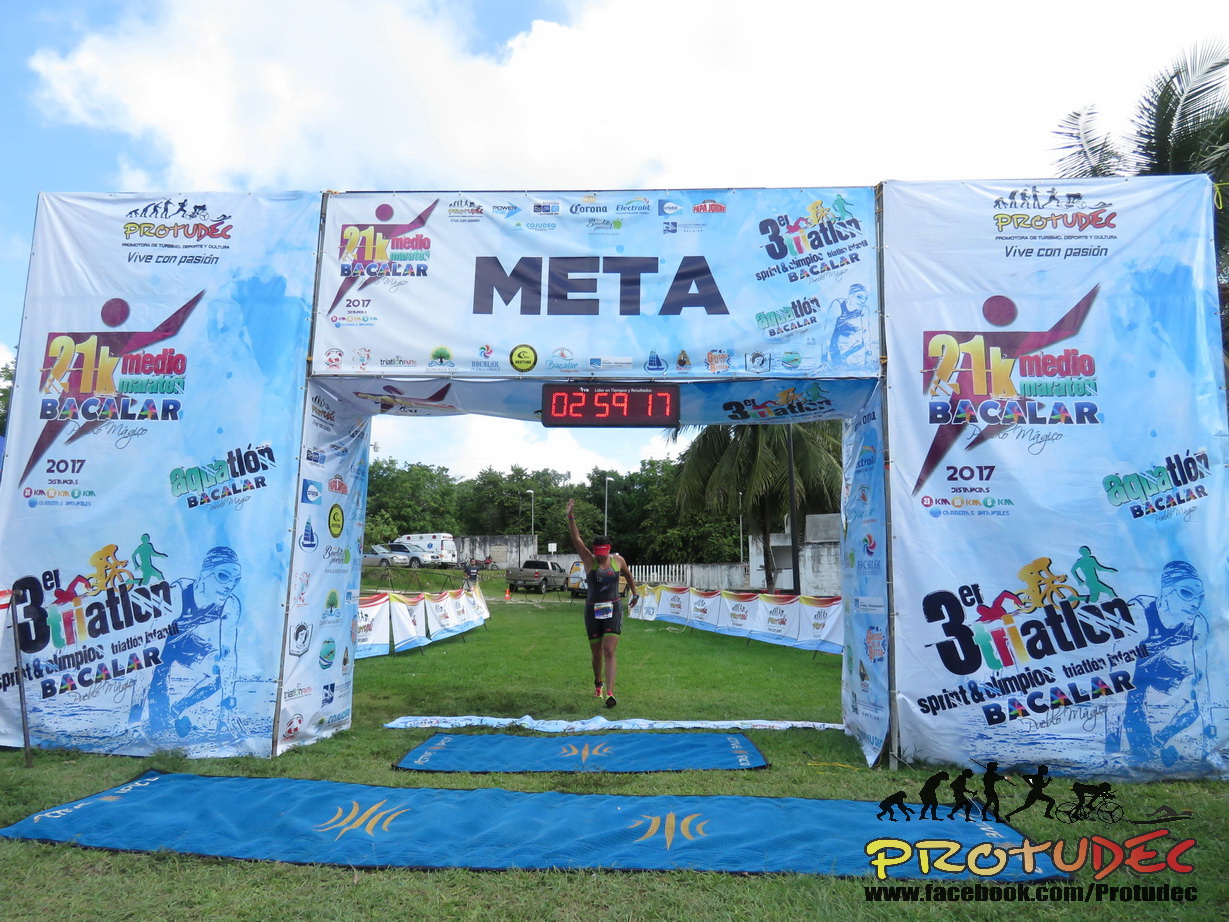A wide rectangular color photograph captures the intense moment of an African-American man finishing a road race. The runner, sporting light brown skin, is prominently centered in the image, approaching the camera with his head facing down and one hand raised in a wave. He is clad in a distinctive black one-piece leotard with green and red accents, complemented by a red visor, and a bib pinned to his chest. Just ahead of him lies a stark white finish line, and beyond it, a large archway constructed from metal tubes, covered in multiple banners.

The most prominent banner, positioned at the top of the archway, reads "META" in bold, dark blue letters on a white and blue backdrop, accented with multicolored details. Beneath this banner, a digital clock exhibits the time "02:59:17" in bright red numbers, marking his race completion. Flanking the archway on both sides are numerous advertisements and graphics, including another notable banner reading "21K MEDEO". Additionally, visible within the scene are a tan truck parked in the grassy background and a wide, rectangular blue towel with intricate gold designs laid out at the bottom of the image. There is also an advertisement depicting a person crouched at the ready, symbolizing the start of a race.